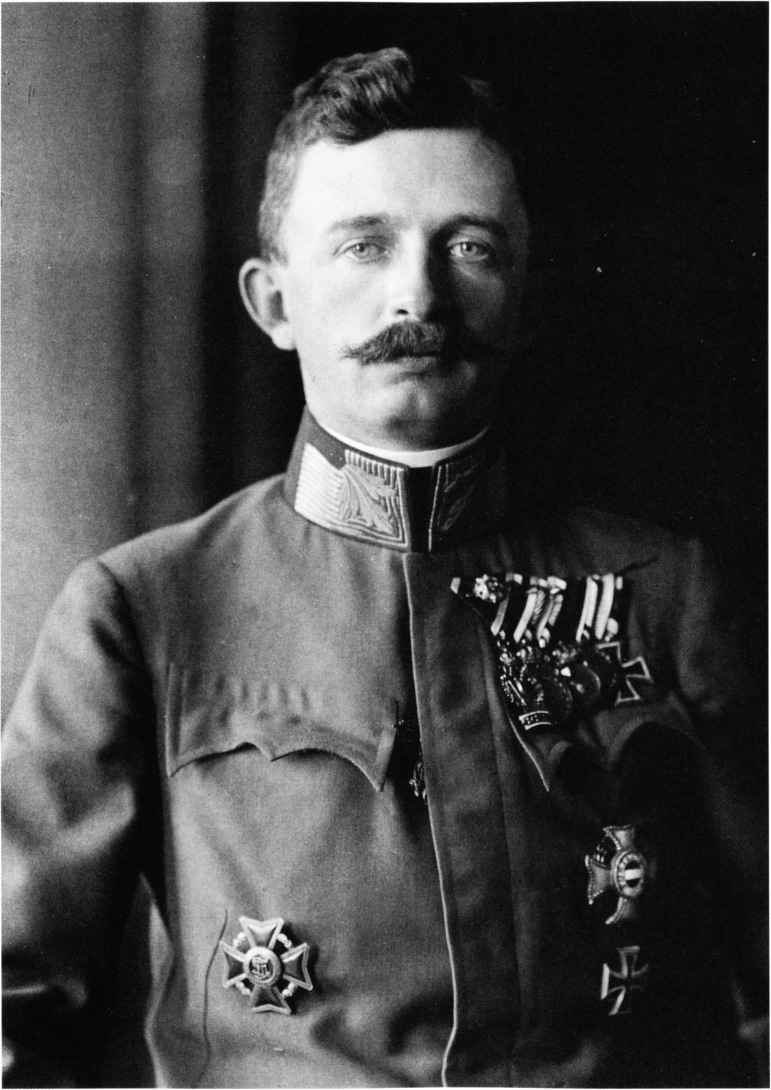This black and white photograph captures a young man in a distinguished military uniform, likely from the early 20th century, possibly around the time of the First World War. His uniform is adorned with numerous medals and symbols, including three on his left chest and a couple of cross-like pins on both sides of his abdomen, perhaps indicative of bravery or heroism. The man stands slightly right of center, facing forward. His dark, medium-length hair is neatly combed back, contrasting with his thick mustache. His ears protrude slightly, and his eyes are light-colored. The high-collared tunic he wears buttoned down the front adds to the formal appearance. Behind him, the background features a curtain to the left and a darker wall on the right, enhancing the solemnity and focus of the portrait. It is suggested that he might be a German soldier, given the style of his uniform and the types of medals displayed.